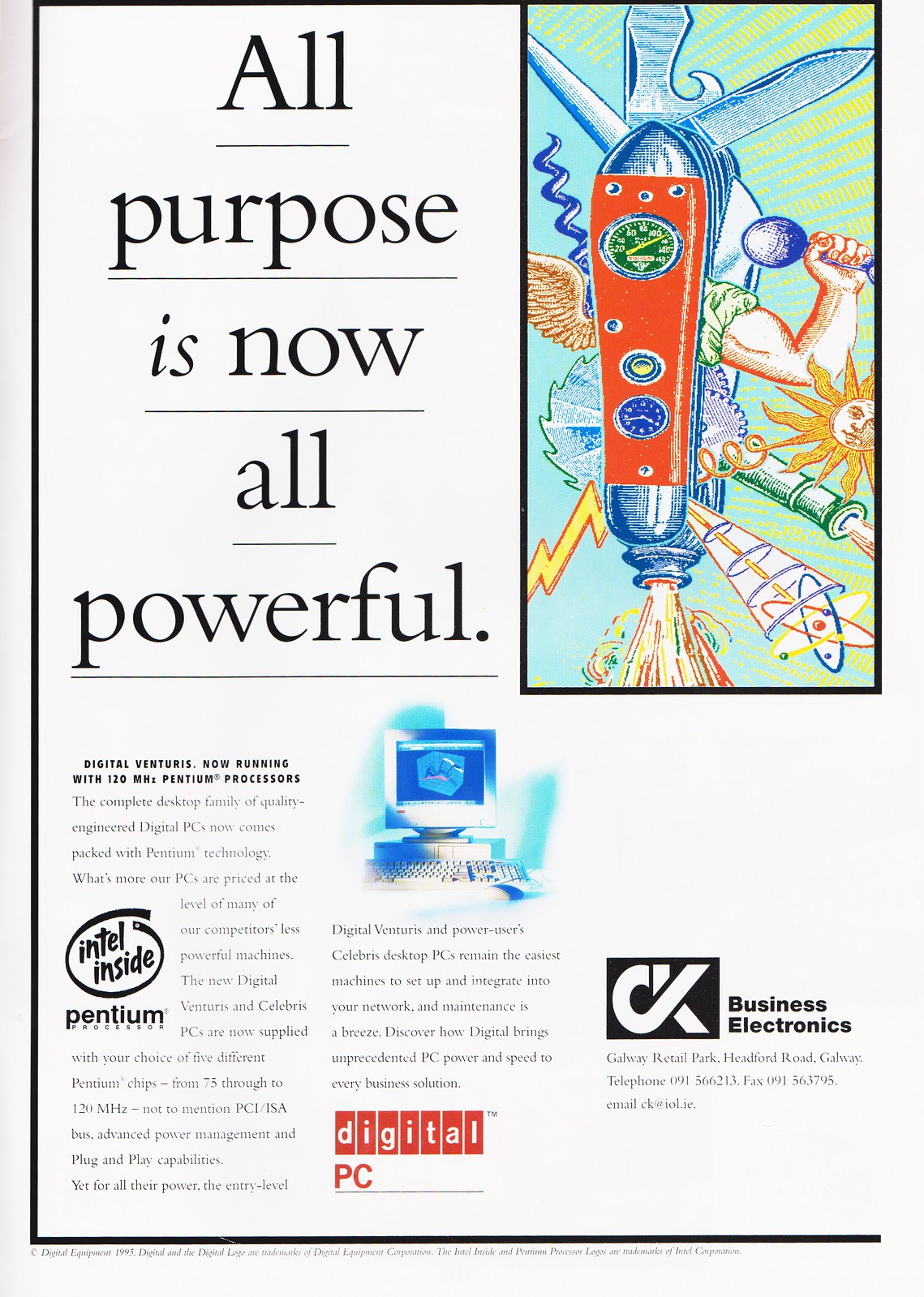The image is a detailed magazine page featuring an advertisement with a white background and a black border. The headline at the top reads "All Purpose is Now All Powerful," with each word underlined and "is" italicized. In the top right quadrant, there is an elaborate illustration of an enhanced multi-tool. This tool includes traditional Swiss Army knife elements such as a corkscrew and box cutter, but also features extraordinary additions like an eagle wing, a lightning bolt, atoms, a human arm holding a microphone, a buzzsaw, and a laser beam, depicted as a "multi-tool on steroids."

The bottom half of the image contains two vertical columns of text elaborating on Digital Venturis and Celebris PCs, which now come equipped with 120 MHz Intel Pentium processors. It highlights the complete desktop family of high-quality, digitally engineered PCs featuring advanced capabilities such as PCI/ISA bus, advanced power management, and plug-and-play, all at competitive prices. The text praises the ease of setup and maintenance, emphasizing the unparalleled power and speed for business solutions.

Adjacent to the columns, there is a striking blue desktop computer monitor prominently displayed in the middle center of the lower portion, while the bottom left corner showcases an "Intel Inside Pentium" logo. At the bottom center, the text "Digital PC" is clearly visible, and in the far right bottom corner, a "Business Electronics" logo is included, reinforcing the advertisement's focus on cutting-edge business technology.